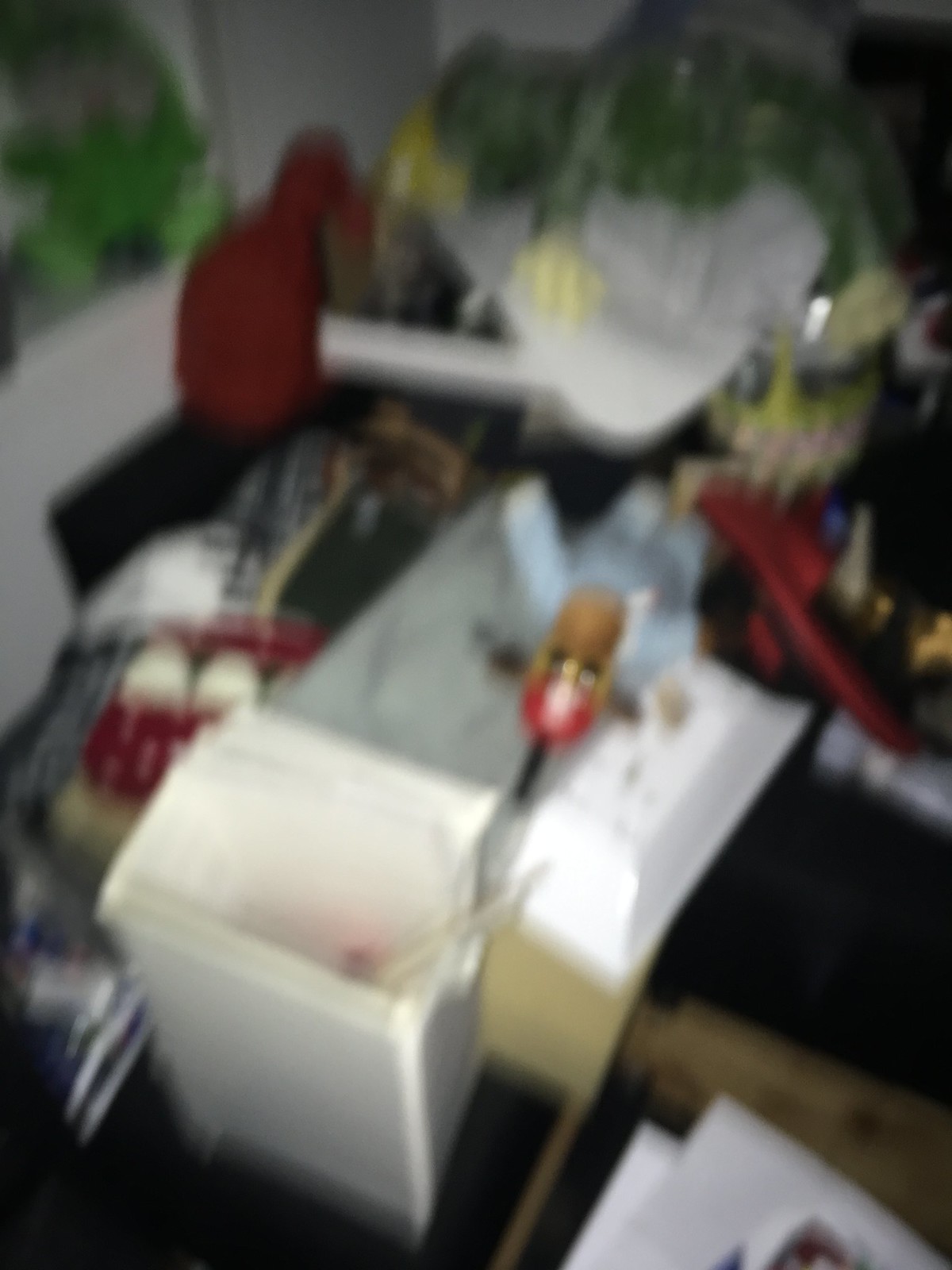A slightly blurry image showcasing a miscellaneous assortment of items scattered on a black couch or bed, accompanied by a matching black ottoman. In the bottom left corner, there's a white container with sticks protruding from it. Adjacent to it is a small wooden doll with a dark stick-like body and vibrant red pants, partially emerging from a box. On the left-hand side, a green, white, and red scarf is draped casually. The right side features a red toy car, and behind the array, a dome housing a small plant is visible. A red bag lies to the left, and the floor beneath is a light brown shade. In the top left corner, nestled in a shelf or shelving unit, is an indistinct green object.